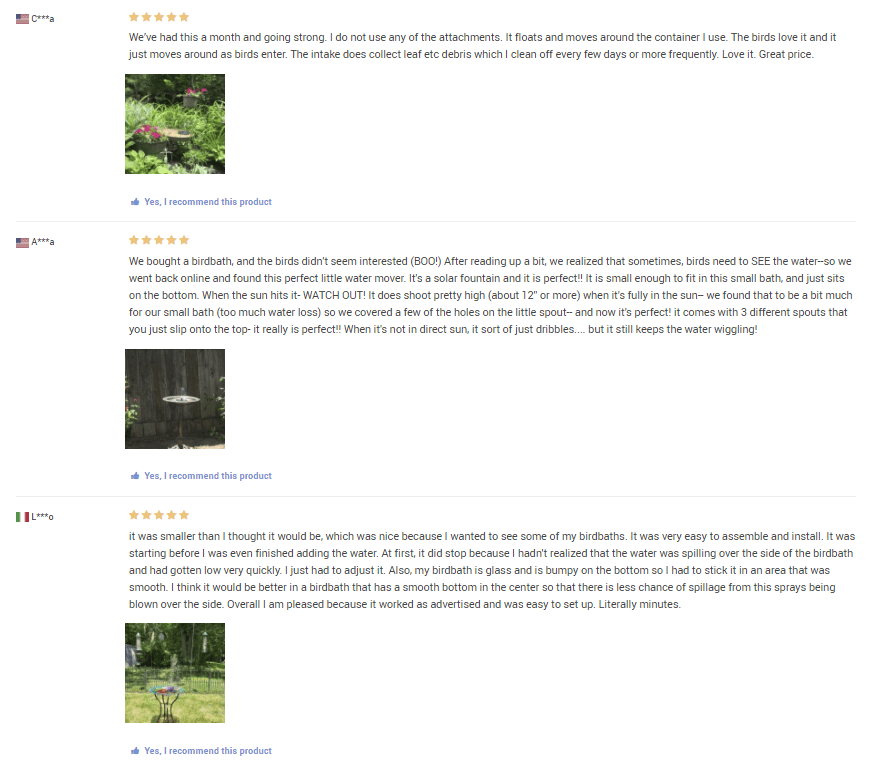Here is a detailed and cleaned-up caption based on the provided information:

---

Screenshot of a website displaying three five-star reviews for a birdbath. Each review features a user’s feedback and begins with a five-star rating. The first review reads, "We've had this a month and going strong. I do not use any of the attachments. It floats and moves around the container I use. The birds love it and it just moves around as birds enter. The intake does collect leaf and other debris, which I clean off every few days or more frequently. Love it, great price." Below each review, there is an image of the birdbath, followed by a thumbs-up icon indicating "Yes, I recommend this product." All three reviews include this recommendation. On the left side of each review, there is a flag indicating the reviewer’s country and a partially obscured username for privacy.

---

This caption provides a clear and comprehensive description of the image and its contents.